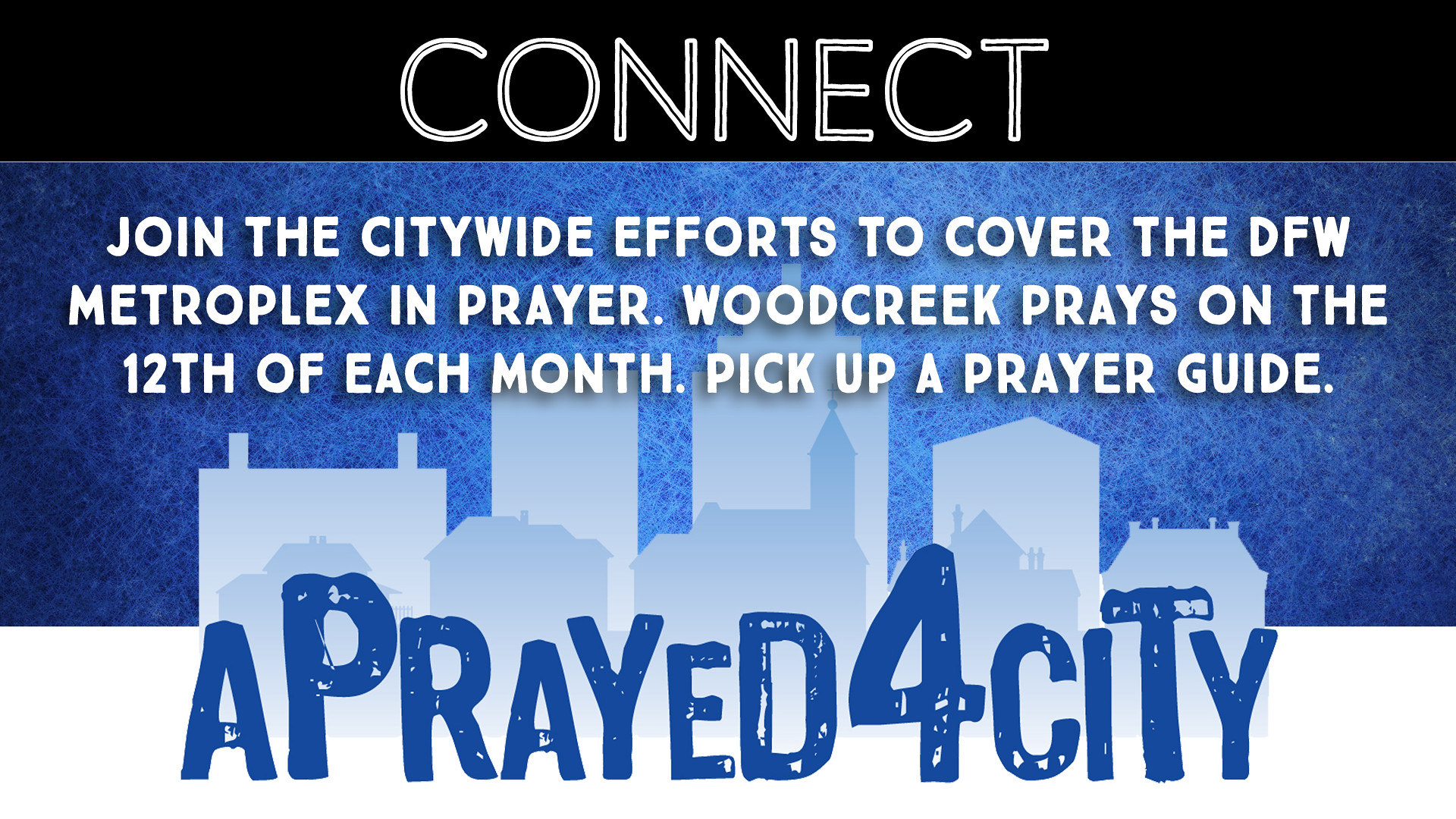The promotional graphic features a sleek horizontal layout designed to catch the viewer's attention. The top of the image has a thin black banner with the word "Connect" in bold white letters. Below this, the main section showcases a deep blue background that transitions from lighter blue in the center to darker blue at the edges, creating a gradient effect.

In the middle of the image, there is a white text overlay that reads: "Join the citywide efforts to cover the DFW Metroplex in prayer. Wood Creek prays on the 12th of each month. Pick up a prayer guide." This text is positioned above a detailed city skyline with buildings in various shades of light blue and white, including homes and a central church. The overall blue color scheme extends to the large text at the bottom, which says "I prayed for a city," rendered in a textured, almost painted style.

This graphic appears to be an invitation or promotional banner for a prayer event, urging participants to join a communal effort and offering guidance on how to get involved. The combination of the detailed cityscape and the text emphasizes unity and community involvement.